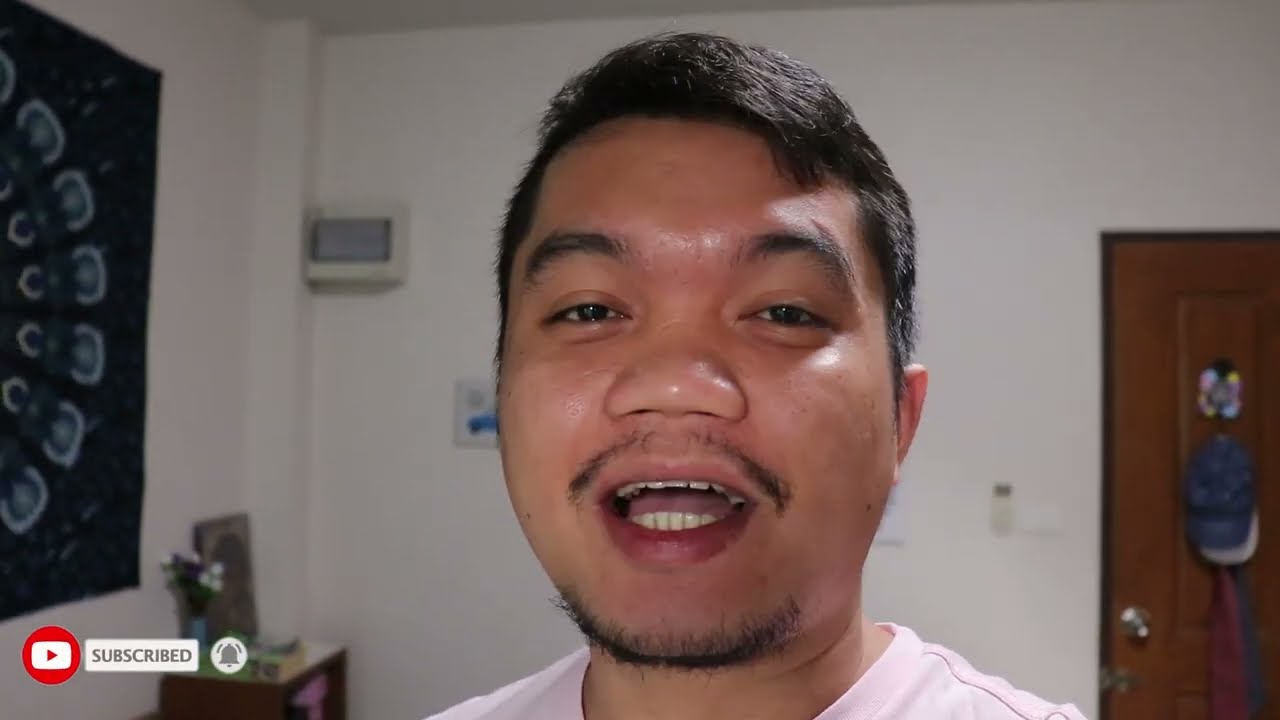The image is a thumbnail for a YouTube video featuring an Asian man with short, dark hair, wide black eyebrows, a wide nose, and a mustache connected to a very short goatee. He is captured mid-speech or mid-song with his mouth open, facing the camera directly. His attire includes a pink t-shirt, and the image is cropped just below his shoulders.

In the background, the room has a white wall with a thermostat visible. Towards the bottom right corner, there is a brown door with two hats hanging on it. On the left side, there is a wall decoration, possibly a black canvas or tapestry with a white or gray decorative pattern, creating a striking contrast. Below this, there is a small chest or table adorned with a vase of flowers and a picture frame.

Additionally, the lower left corner of the thumbnail features a red and white YouTube logo next to a rectangular white "SUBSCRIBED" button, and a circular icon with a bell, indicating that this is a YouTube video thumbnail.